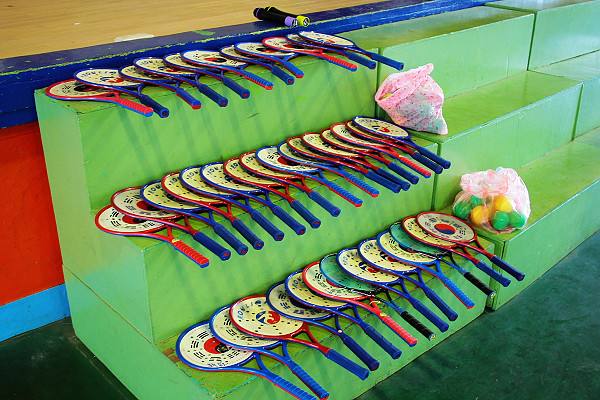The image depicts a green staircase made of wood, with three steps resembling seating, set within a sports warehouse. Various types of rackets are organized in three rows on these steps, stacked horizontally. The rackets display a range of colors including blue, red, black, and some with intricate designs and flat surfaces lacking traditional strings. There are about 10 or more rackets per row. Adjacent to the rackets are two pink plastic bags containing an assortment of green and yellow balls. The background features panels in blue, red, and light blue colors, with a dark gray floor adding contrast to the vibrant setting.